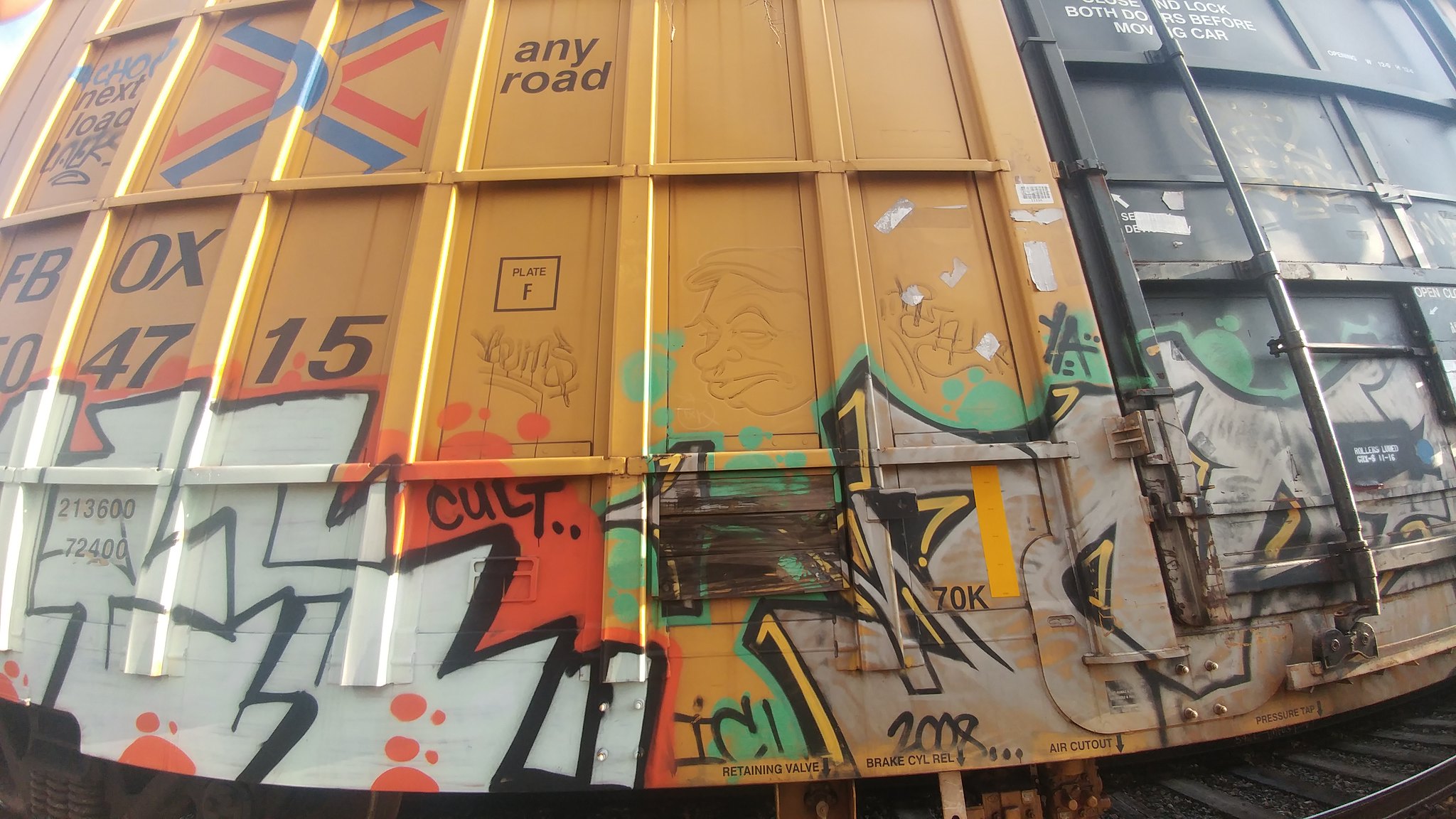The image showcases a horizontally-oriented, wide-angle photograph of a cargo-hauling rail car, highlighting detailed elements of the car and the surrounding area. The view is slightly distorted but captures a side angle of the rail car. At the far bottom right, part of a silver rail track with dark grayish wooden ties is visible, flanked by a gray metal pipe running along the background. The rail car’s surface is made of corrugated steel panels, with imperfections emphasized by the lens distortion. The car’s base color is a brownish-yellow, with a significant amount of graffiti.

On the upper section of the rail car, distinct markings and graffiti are prominent. The words "Any Road" are clear, followed by the identification numbers FBOX04715. To the top left, two crisscrossed arrows, one red and one blue, are notable. There’s a large amount of randomly spray-painted graffiti, with some discernible pieces like the word "CULT" in black, near orange spray paint, and the year 2008. The car also features black block letters I, C, L, and various other graffiti elements, creating a chaotic visual.

A notable grid of vertical rectangles adorns the side of the car. The first rectangle states "Next Load" in black lowercase font, followed by the aforementioned arrows. The successive rectangles provide further information: "Any Road" spelled out, the letters FB, the partial number "47," and more identifying marks partially obscured by graffiti. The lower sections of the rectangles showcase varied graffiti, including white, black, and orange hues with scribbled black lines; some portions display numbers like 213600 and 72400.

Additionally, there is a black door with a latching mechanism on the right side of the image. The entire scene is set against a backdrop with sporadic pebbles seen between the rail tracks, blending industrial utility with an urban canvas of street art.